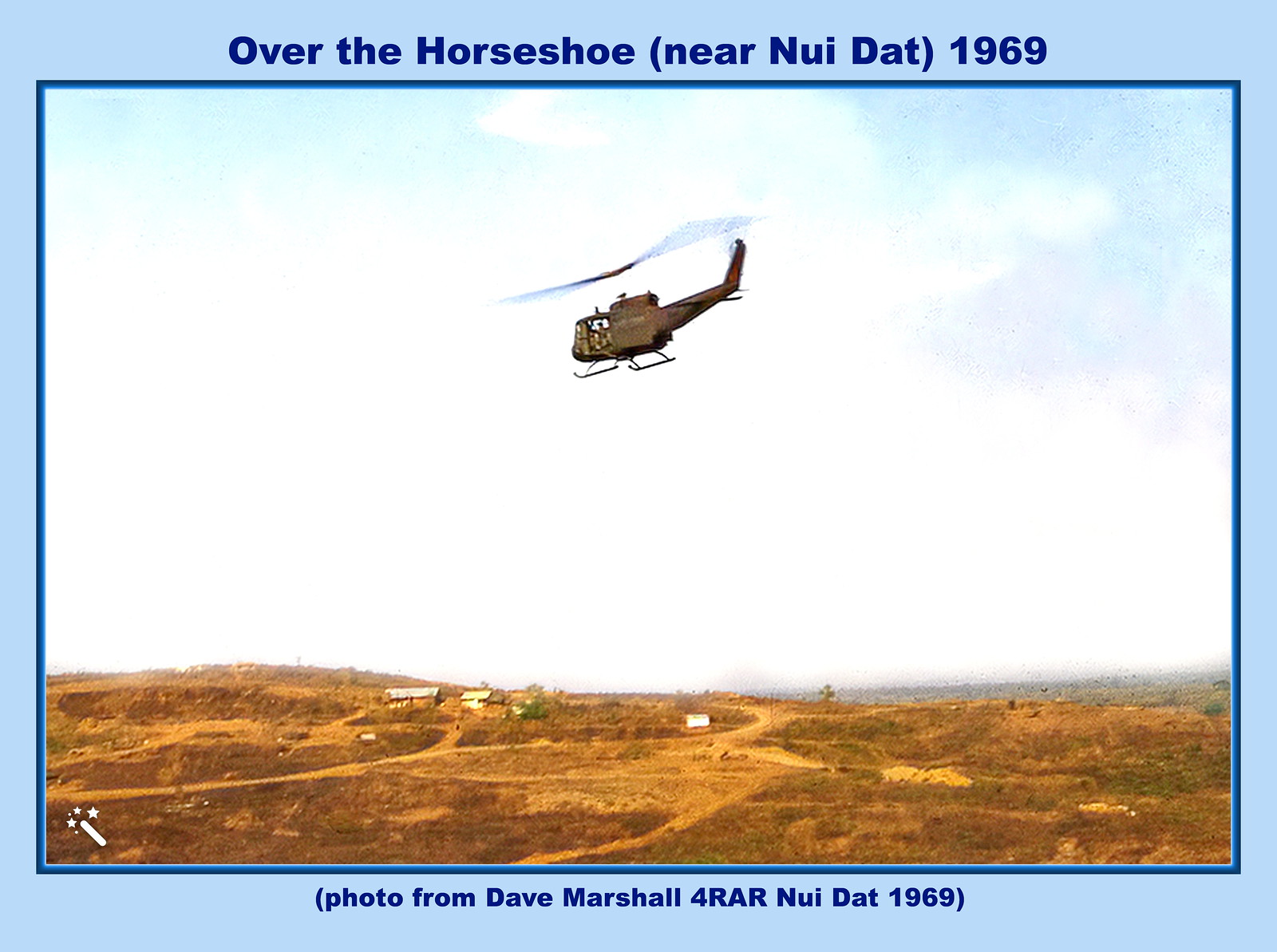The photograph features a rugged, brownish-green helicopter flying over a sparsely populated, desert-like landscape with a few scattered buildings and dirt roads. The land below appears brown and arid, with low brush and no trees, while the sky above is mostly filled with clouds, though a hint of blue sky peeks through. The image is bordered by a blue and a lighter blue frame, with the text "over the horseshoe near Nui Dat 1969" in dark blue font at the top and "photo from Dave Marshall for RAR Nui Dat 1969" at the bottom, indicating its historical context.